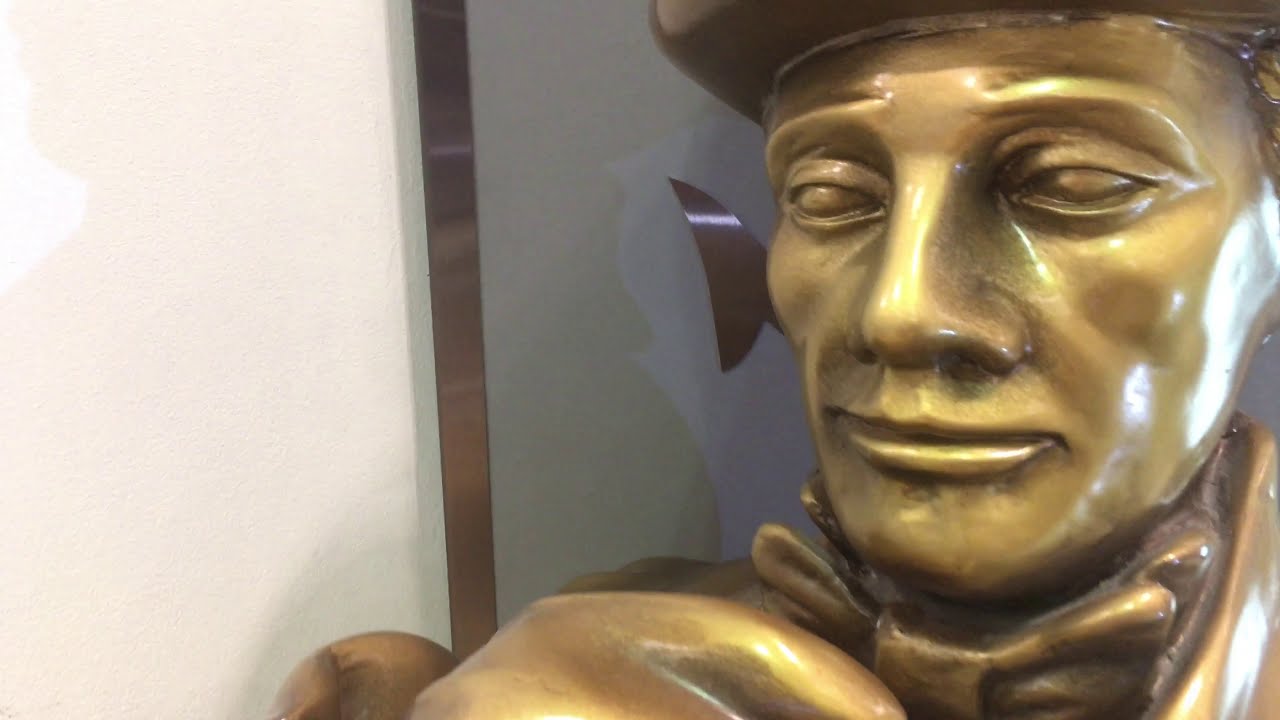A rectangular, full-color photograph taken indoors showcases a golden statue of a male figure prominently positioned in the center. The background features an off-white wall, which casts shadows due to a light source from the right side of the image. This light accentuates the statue's facial features, including a large nose and open eyelids without pupils, revealing gold bulges instead of eyes. The statue is attired in a high-collared jacket with a fluffy shirt, giving it a detailed and textured look. While its hat is not fully visible within the frame, the statue's raised hand appears to be adjusting a bow tie on its neck. To the left of the statue, part of a bronze-framed mirror can be seen hanging on the wall. The overall ambiance suggests that the photograph might have been taken in a museum or a gallery setting.